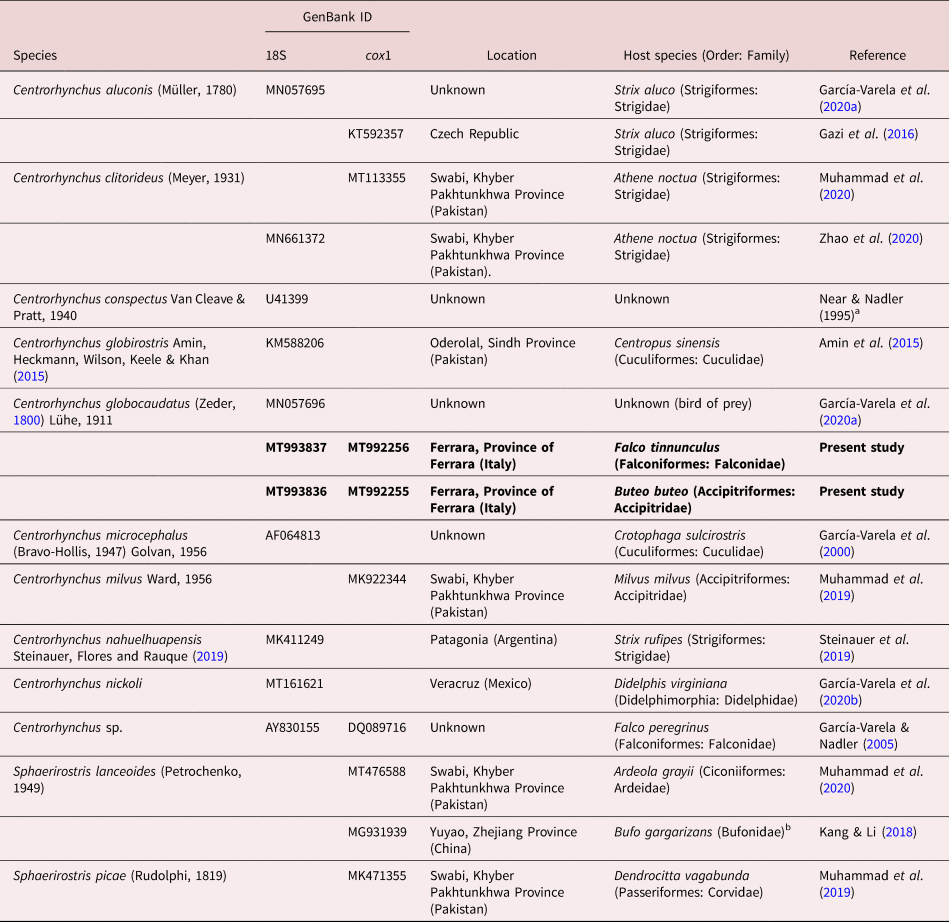The image showcases a detailed scientific chart on a light pink background, filled with meticulously organized data in various columns. Each row catalogues different bird species with their full scientific names and respective GenBank IDs (divided into 18S and COX-1). The table includes columns titled 'Species,' 'GenBank ID,' 'Location,' 'Host Species (Order Family),' and 'Reference.' The locations listed range from the Czech Republic and Romania to Swabi and Veracruz. Host species names, such as Strix Aluco and Centropus Sinensis, are in Latin. References are cited in blue text with names like Garcia Varela et al. and Muhammad et al., standing out. The small text and numerous columns make the chart comprehensive but densely packed with valuable data, akin to a page torn from a scientific textbook.